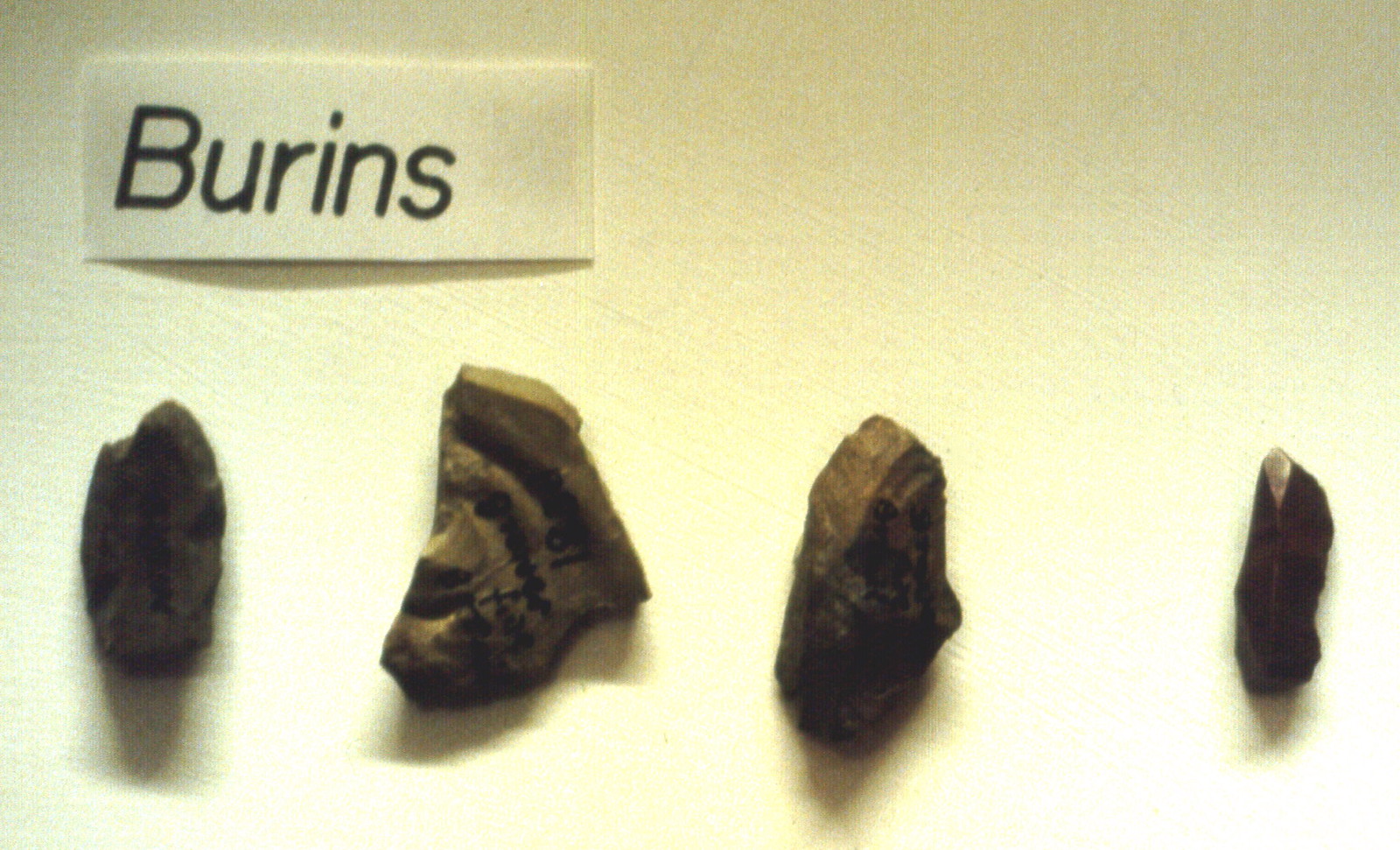The photograph features four distinct, dark-colored rock pieces arranged horizontally on a slightly textured yellow-beige background. At the top left corner of the image, there is a small white rectangular piece of cardboard labeled "B-U-R-I-N-S" in black lettering. The rocks vary in size and shape but share a rough, aged texture, suggestive of ancient artefacts or fragments.

The first rock on the left is narrow and oblong with uneven edges, casting a slight shadow. The second rock, the largest among them, has a more irregular shape with prominent grooves that almost appear to form a face, including what looks like a round, circular nose in the middle. The third rock is slightly larger than the first, showcasing a distinct rigid area and dark coloring at the bottom. The fourth and smallest rock is dark with a teardrop-shaped white mark at its top. Each rock's unique shape and texture, combined with the shadows they cast, enhances their ancient and weathered appearance.